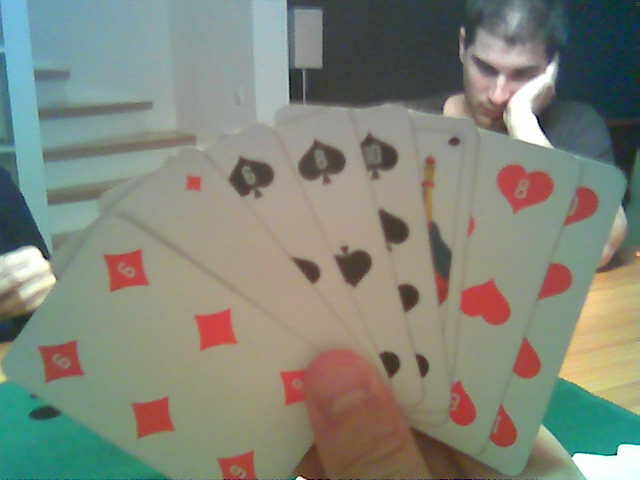In the foreground of the color photograph, a hand holding a fan of playing cards dominates the composition. The thumb protrudes into the frame from the bottom, partially covering the lower edge of the spread cards, which include a six of diamonds, an ace of diamonds, a six of spades, an eight of spades, a ten of spades, an unidentifiable face card (likely a spade), an eight of hearts, and a partly obscured nine or ten of hearts. The cards, though slightly out of focus, are the central element of the image.

The scene is set on a green table, with a hint of a cardboard floor visible in the lower right corner. Behind the card-playing hand, the upper right section of the photo reveals an opponent—a man with dark brown or black hair dressed in a black t-shirt. He leans his left elbow on the table, resting his head in his hand, appearing deep in thought. On the far left edge of the image, a sliver of another player is discernible, displaying only a portion of their arm and hand, also clad in black.

In the background, the top left corner features a staircase with white-painted walls framing the wooden steps and white risers. Adjacent to this, a darker area suggests another room, partially illuminated by a square-shaped lampshade sitting on a table or floor lamp, adding a touch of understated domesticity to the scene.